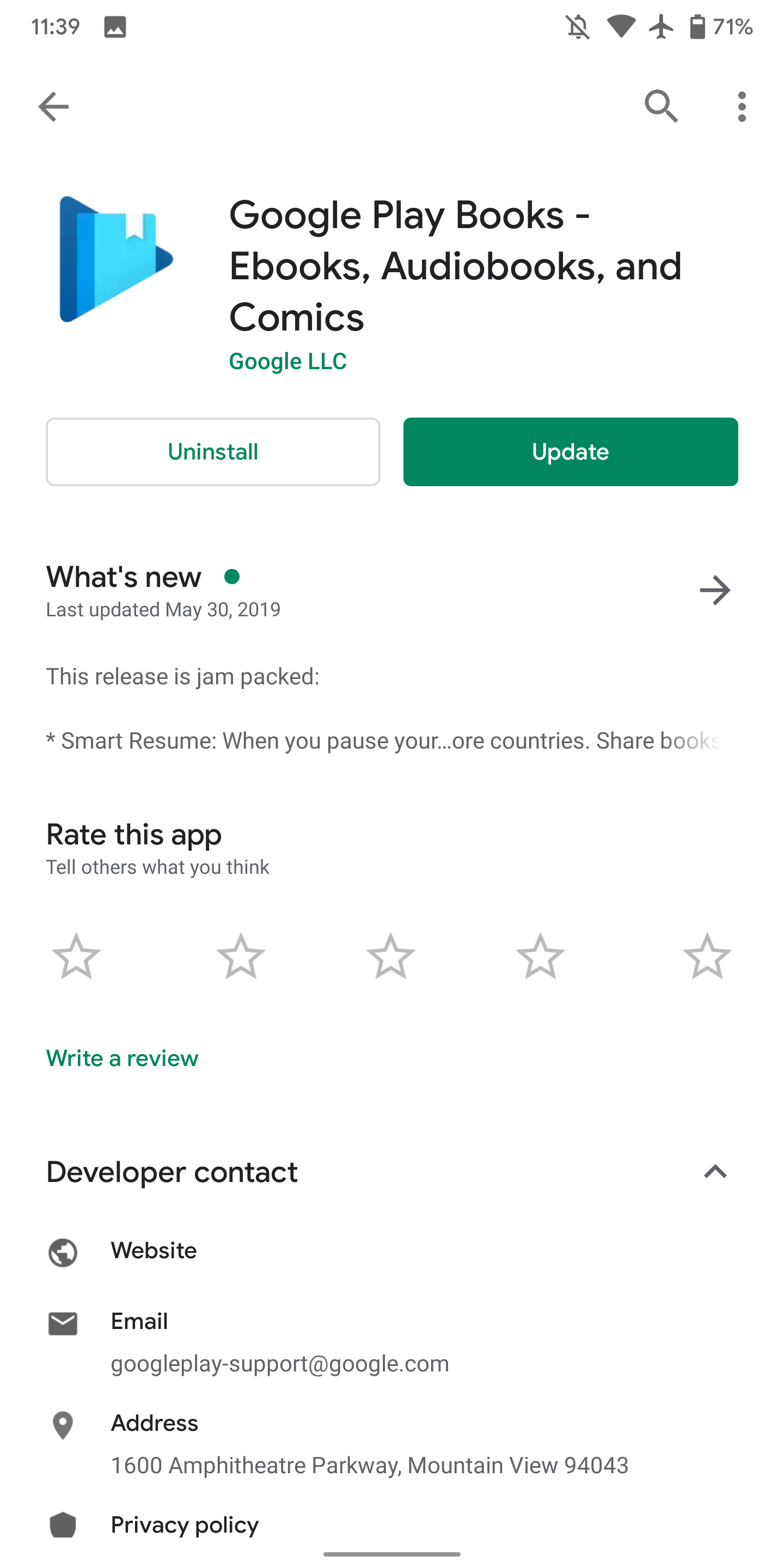This image is a detailed screenshot of the Google Play Store page for an app. The rectangular screenshot captures a variety of elements typical to a mobile device's interface. 

In the upper left corner, the time reads 11:39, while the upper right corner displays several status icons, including a battery bar that is approximately two-thirds full and shows the percentage "71%". 

Beneath the status bar, the app icon is prominently displayed. This icon features a rightward-pointing triangle with a book in its center, colored in shades of dark and light blue. 

Next to the icon, the app's title is written in bold black text: "Google Play Books: eBooks, audiobooks, and comics". 

Directly below the app title, there are two buttons: one on the left with a white background and green text reading "Uninstall," and a second button with a dark green background and white text reading "Update".

The section titled "What's New" follows, detailing the app's recent updates in black text. 

Further down, a "Ratings" section appears with five outlined gray stars, indicating where users can rate the app. Underneath the stars, a green link invites users to "Write a Review."

At the bottom of the screenshot, there is information about the developer, including options to visit the website, send an email, or review the app's privacy policy.